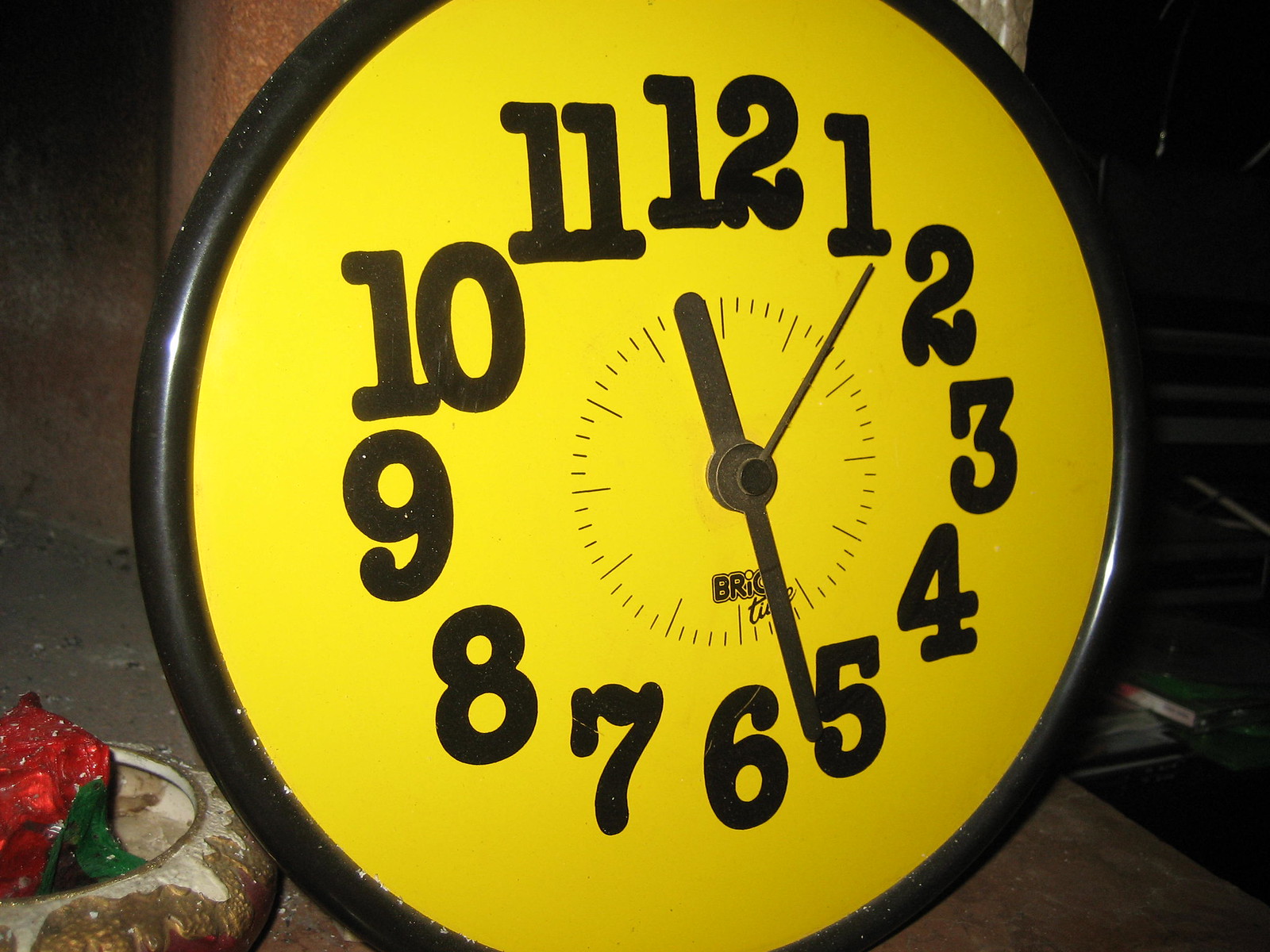In this real-life photograph, a large circular clock stands propped up against an indistinct background. The clock features a prominent black tubular frame with a rounded shape. The clock face itself is a vivid yellow, adorned with large black numerals from 1 to 12 encircling it. The clock's metal hands, appearing dusty or dirty, indicate a time of 11:25, with the seconds hand positioned between the 1 and the 2. The clock's inner circle is marked with small dashes representing minutes and longer dashes at each hour.

A logo reading "BRIC" is situated just above the 6, partially obscured by the minute hand. Surrounding the clock is an enigmatic scene dominated by rusty, metallic, and cement surfaces, giving a starkly industrial feel. These surfaces, covered in reddish-brown hues and what appears to be debris, suggest a neglected or abandoned area.

In the bottom left of the image, there is a crusty and dirty bowl containing what looks like a red and green wrapper. The background on the right is shrouded in darkness, making it difficult to discern details, yet there are faint hints of lines that might be pipes or other industrial structures. The overall ambiance of the photograph is one of decay and disuse, lending a gritty authenticity to the scene.